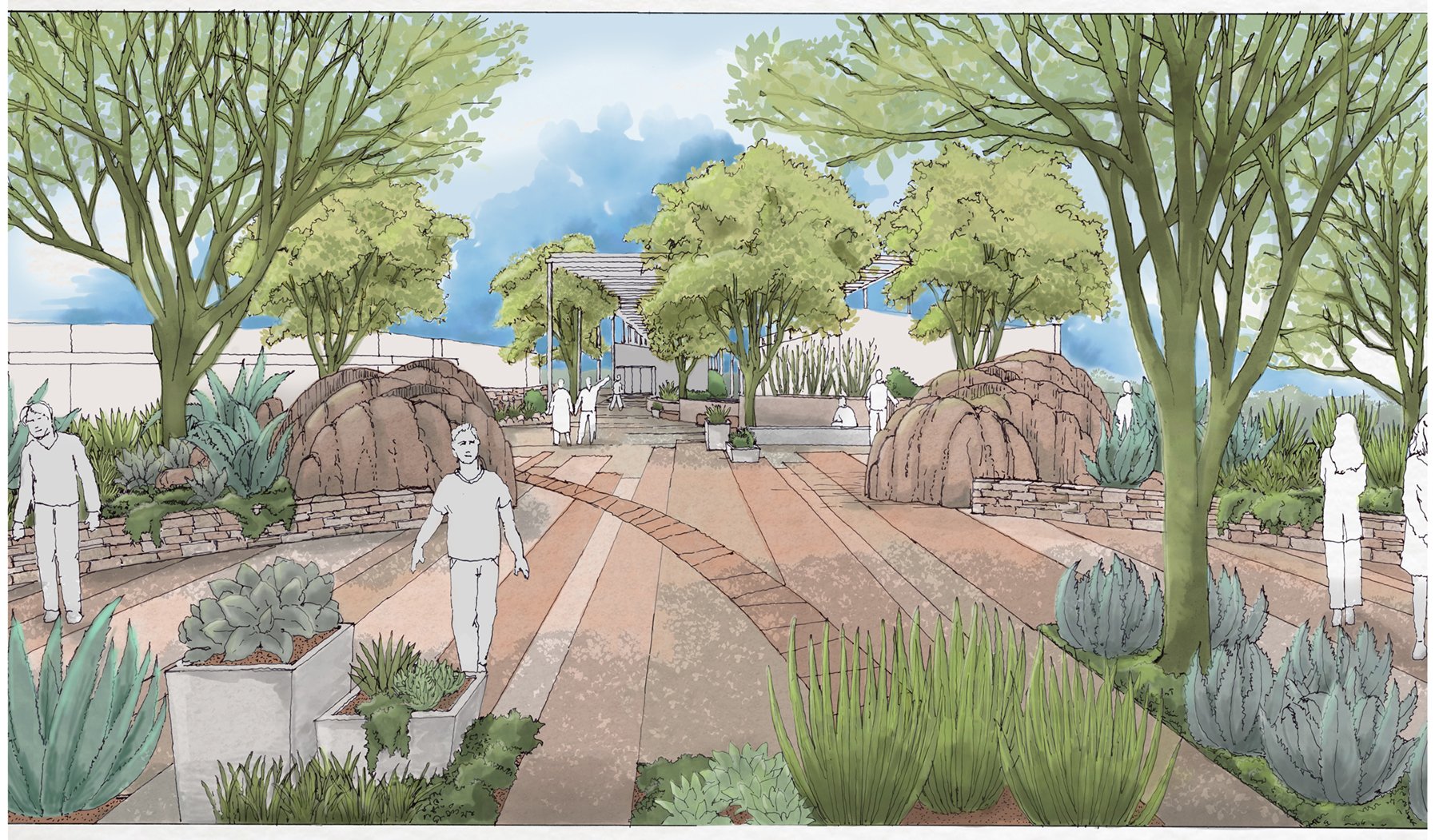This watercolor artistic rendering depicts a serene garden or park, possibly within hospital grounds. The composition features a blend of natural and architectural elements, with straight and curving stone pavers creating a broad walking space. The sky transitions from light blue to a darker shade near the building in the background, which is partially covered by a sunshade or pergola.

The lush greenery includes a variety of succulents, cacti, and trees, often contained within concrete planters and raised beds. Additionally, large boulders are strategically placed to enhance the visual interest of the landscape. 

Human figures in the scene are depicted as simplified white silhouettes with black outlines, standing in stark contrast to the colorful environment. There are several individuals throughout: one person to the left gazes outward, another man stands prominently in the middle foreground, two women on the right examine the plants, and a man sits on a planter in the back. Another key feature is a couple walking together, further enhancing the tranquil and communal atmosphere of the space. Each detail harmonizes to create a cohesive and inviting outdoor environment.